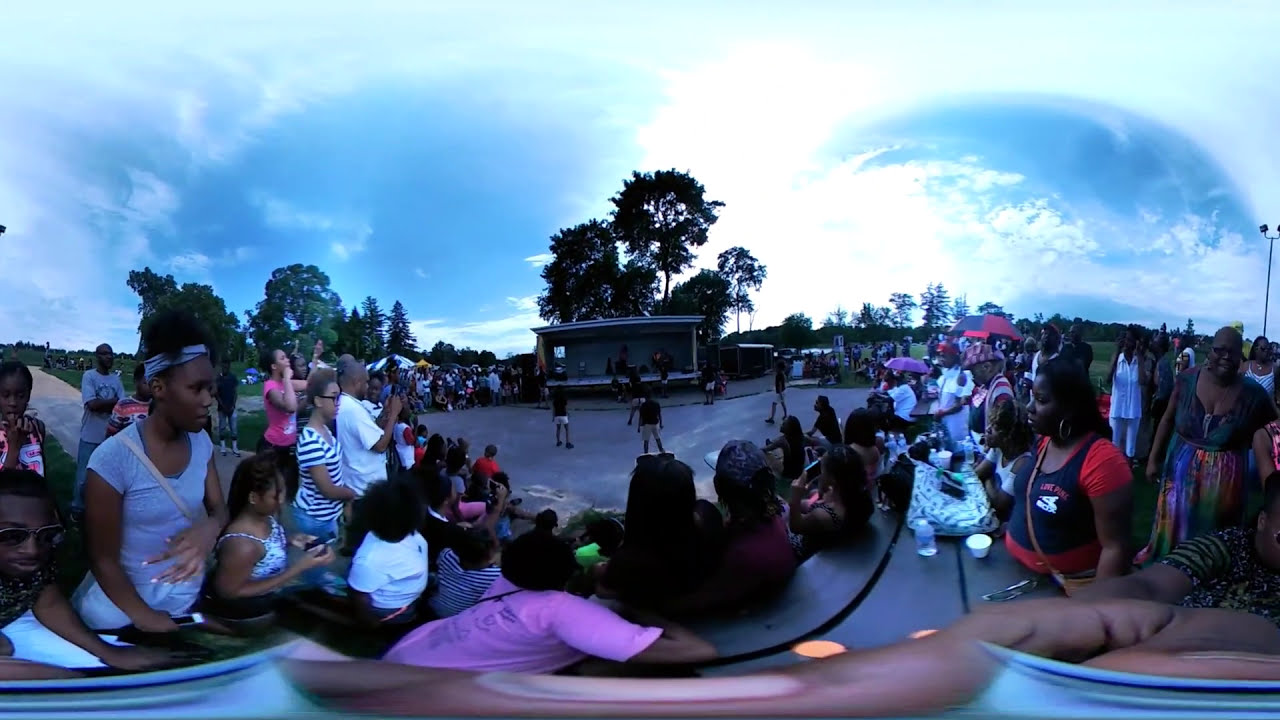The image captures an outdoor scene in a park, filled with a large, diverse crowd of men, women, and children gathered around an amphitheater. The sky above is a vibrant blue dotted with puffy white clouds, with the sun shining brightly, casting light across the scene. The park is surrounded by lush green trees that frame the image beautifully. In the center, there's a small concrete rectangle where several young men in black shirts and shorts appear to be engaged in a game or performance. A built-up stage with a roof and fog lights mounted on a large metal stand is also visible in the background, drawing the attention of many spectators. Some audience members are sitting on tiered stands or steps, while others are milling about, holding up cameras or simply observing the scene. On the left and right sides of the image, you can see grassy areas and more people seated, along with a glimpse of the fields beyond the crowd. The panoramic shot also captures part of the photographer’s thumb at the bottom and a partial view of a woman wearing a patterned short-sleeved top and glasses on the right edge.